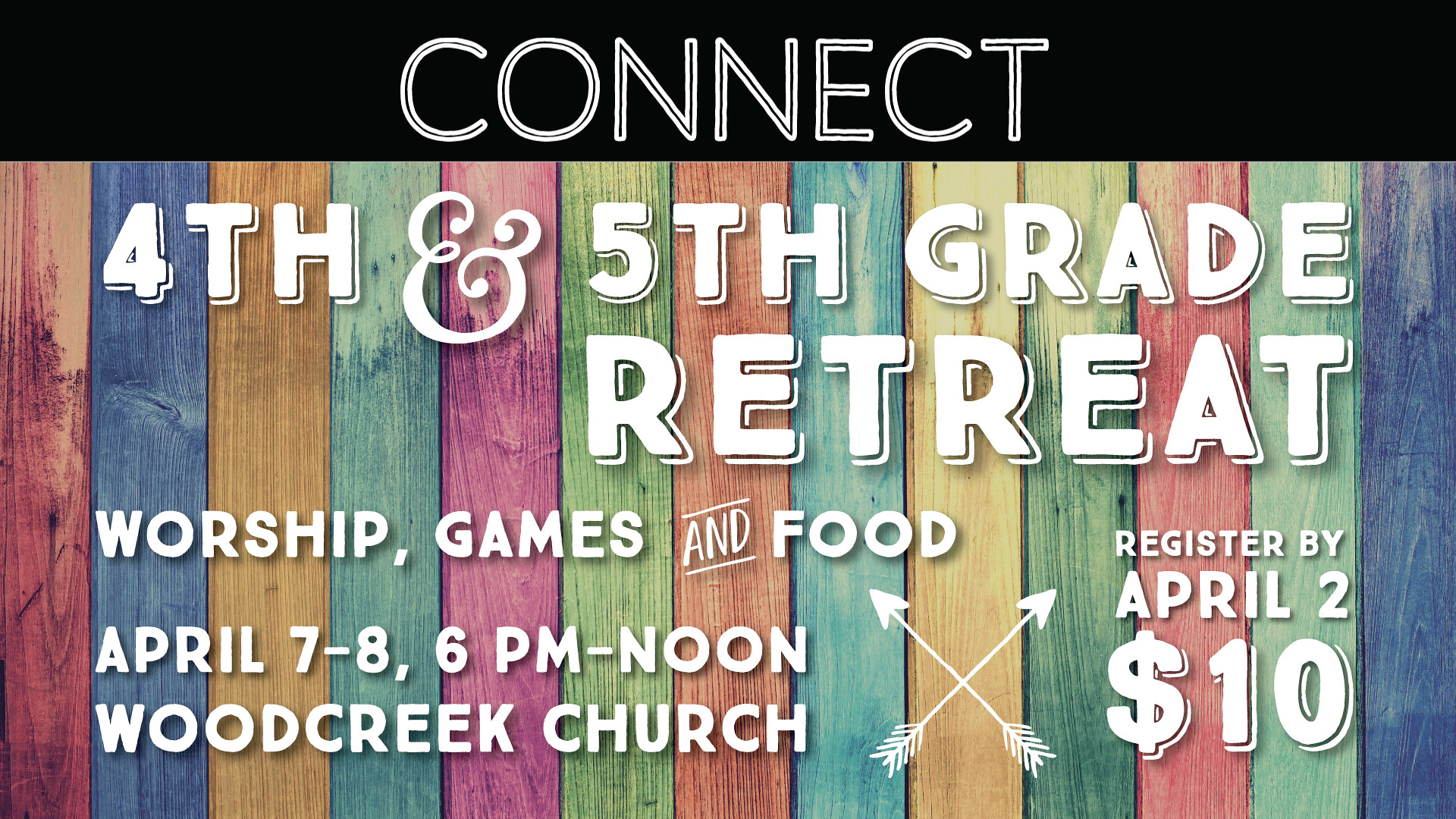**Flyer Description:**

The vibrant flyer for the upcoming event features a large banner at the top reading "Connect" in bold white letters set against a sleek black background. Below this, the main announcement details the "4th and 5th Grade Retreat" in prominent white letters. This section is superimposed over a colorful wooden fence background with vertical slats painted in alternating hues of red, blue, orange, green, pink, yellow, and more, giving a lively and inviting feel.

Additional information is elegantly laid out: the event promises "worship, games, and food" and is scheduled for April 7th through 8th from 6 PM to noon at Wood Creek Church. 

In the center of the flyer, two white arrows intersect to form an X, creating a dynamic focal point between the details on the left and right sides. On the right, attendees are reminded to "register by April 2nd," with a fee of $10 clearly noted.

The overall design combines a rustic charm with a modern aesthetic, providing clear and inviting details for this engaging and fun-filled retreat.